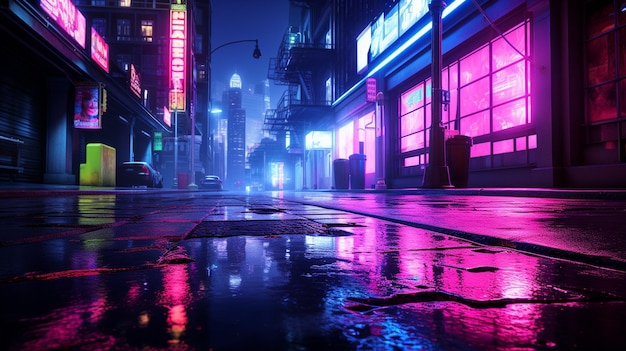This digital photo depicts a vibrant, rain-soaked city street at night, resembling a still from a video game due to its vivid and stylized details. The scene is devoid of people, suggesting it was taken very late at night or early in the morning. Tall buildings flank the street, with a large illuminated structure looming at the end of the road. The wet pavement brilliantly reflects the array of colors emanating from various sources, including windows and neon signs, casting blues, light blues, pinks, and greens onto the surface. On the right side of the street, a building glows with a blue neon sign and pink-lit windows, while the left side features signs and advertisements, possibly for a hotel or food establishment. A rectangular billboard with unreadable foreign letters hints at an international setting. A couple of cars are subtly parked along the road, and trash cans in an alley contribute to the urban atmosphere. The overall mood is mesmerizing, enhanced by the reflective wet ground and the kaleidoscope of colors, creating a scene that feels both real and fantastical.